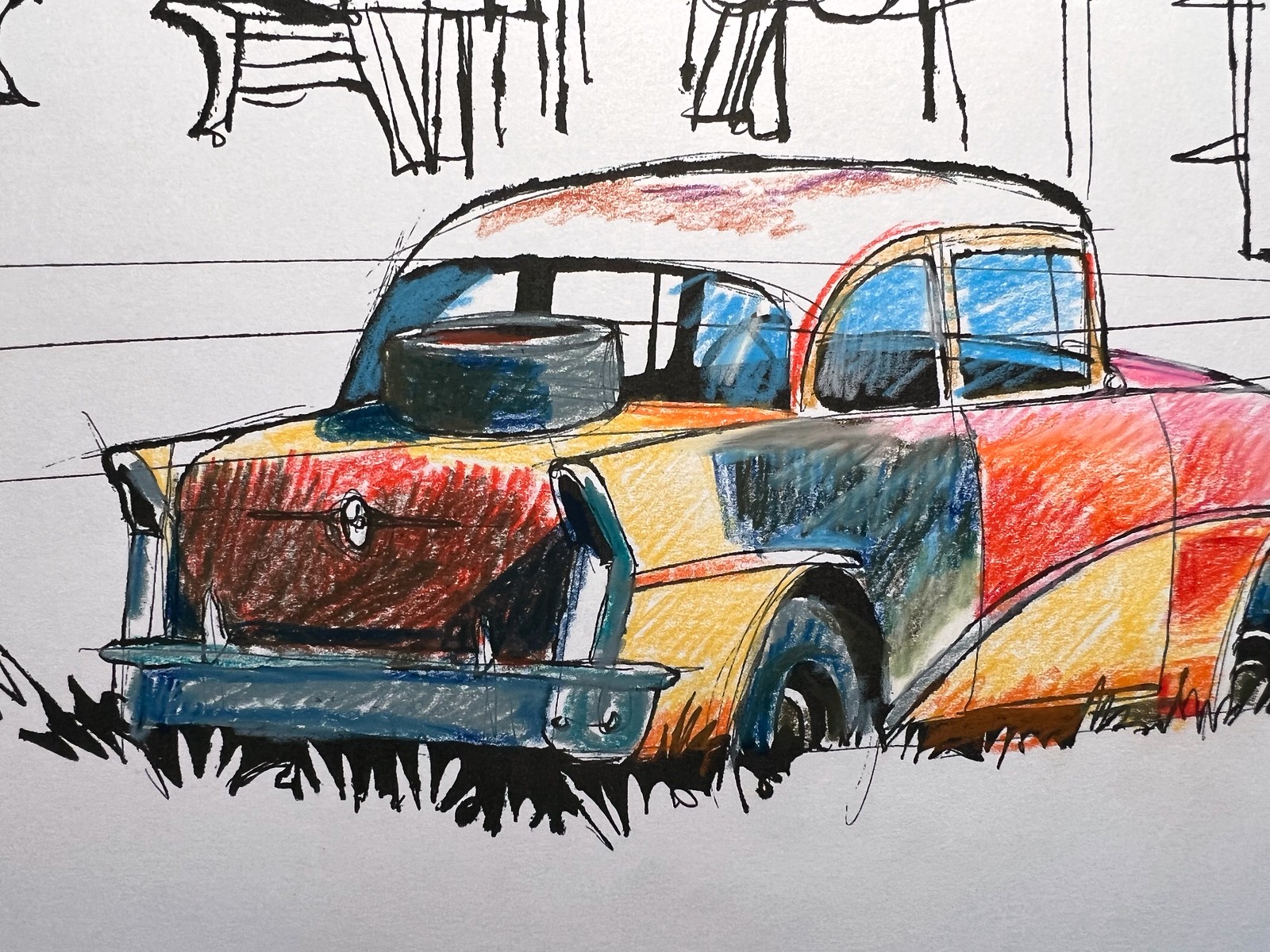This detailed sketch depicts an old, multi-colored car positioned on a grassy surface. The sporadic black grass outlines enhance the unique, hand-drawn texture of the scene. The car's roof is predominantly white, but streaks of purple and reddish hues, reminiscent of crayon strokes, add an artistic flair. At the rear, a distinct black tire rests on the trunk, which is adorned with an orange and blue palette. The tire itself features a mix of black, blue, and gray shades. The vehicle's overall appearance is a vibrant blend of orange, red, black, and blue, creating a striking and colorful visual. In the background, there is an indistinct design or text, subtly framing the car and adding an element of intrigue to the composition.